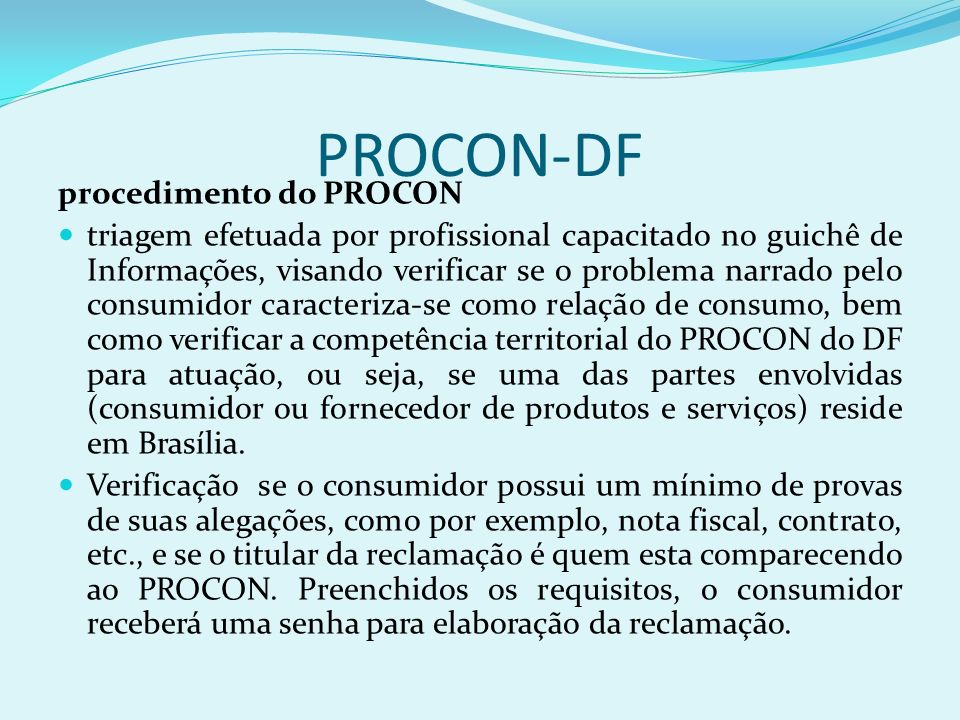The image is a text-based slide with a predominantly light blue background and a darker blue wavy pattern at the top. At the very top of the slide, in all capital letters and dark blue color, it reads "PROCON / DF". Below this header, there is a line of bold black text that states "PROCEDIMENTO DO PROCON". Underneath, there are two bullet points, each represented by small aquamarine blue circles. The text next to the bullet points is extensive and written in Portuguese, indicating detailed procedural information likely related to consumer protection in Brasília, Brazil. The text in the bullets covers the professional capacity required, consumer issues, and necessary documentation such as fiscal notes and contracts. The slide seems to be part of a presentation, providing an in-depth breakdown of the procedural aspects governed by PROCON.